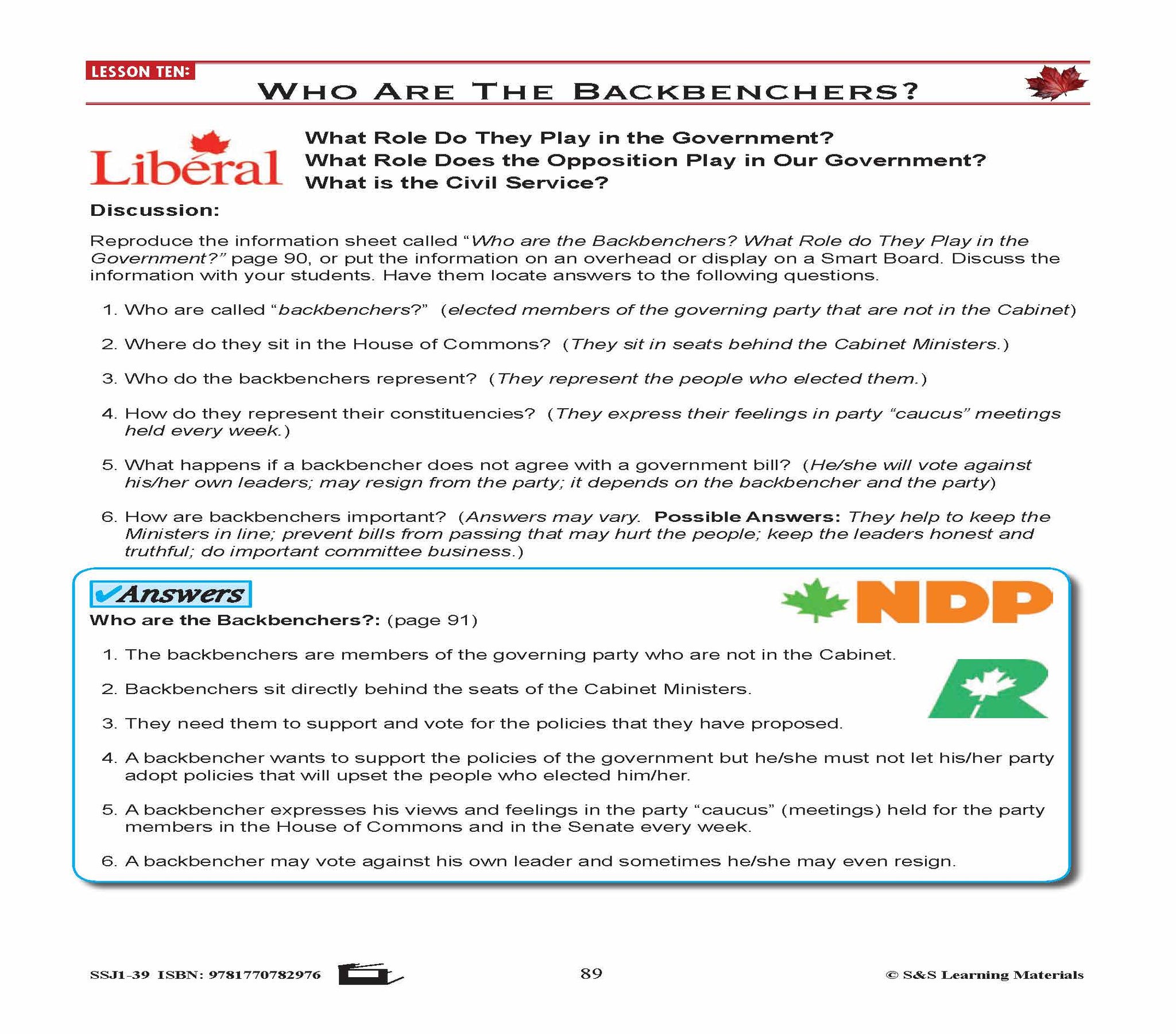This image depicts a page from a pamphlet or book, specifically Lesson 10, with the title "Who are the Backbenchers?" prominently displayed in black text on a white background. In the upper left corner, the white text on a red background reads “Lesson 10” and in the upper right corner, a red maple leaf symbol is present. Below the title, a red line separates the header from the main content. There are several sections addressing key questions and answers, including discussions on roles within the government, the opposition, and the civil service. The questions section features six inquiries about backbenchers, such as their role, seating in the House of Commons, representation, and importance. The answers are presented in black text on a blue background, with the label “answers” marked with a blue checkmark. An additional box in the lower section includes black text on a blue background stating "Who are the Benchmarkers?" alongside another maple leaf, this time integrating an NDP symbol with a maple leaf at the center. The page appears geared towards facilitating classroom discussions, with mentions of potential display methods like overhead projectors or smart boards, and the content is reproduced for educational purposes.